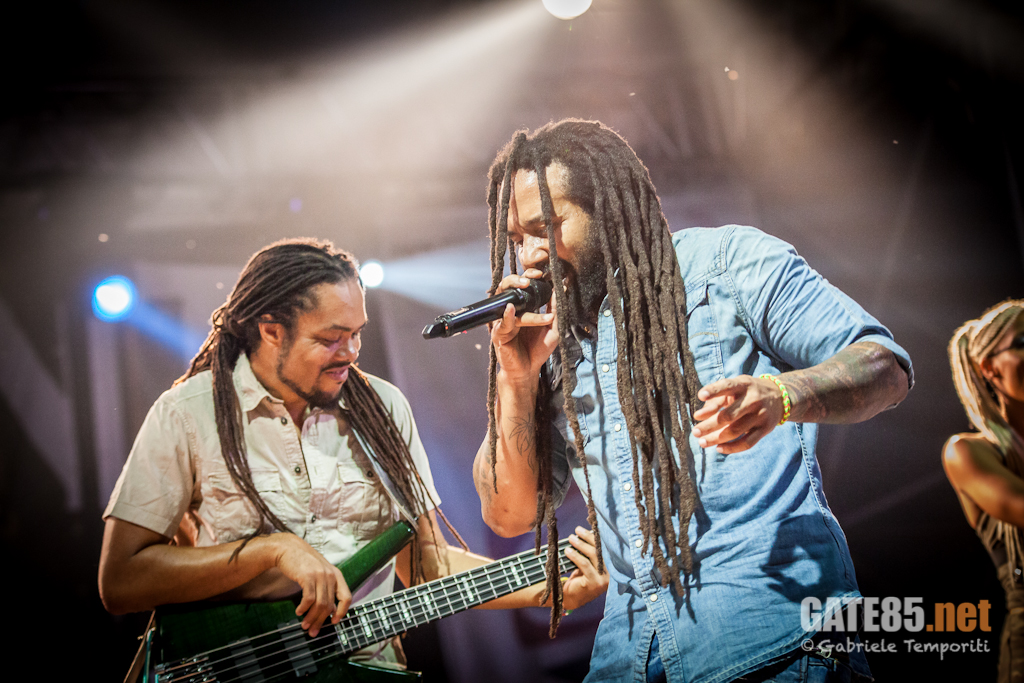In this vibrant image, at the center, a male musician with long brown dreadlocks passionately sings into a black microphone, his left hand extended expressively. He is clad in a light blue denim button-up shirt. To the left, barely visible off-screen, is a female with long hair. On the right stands a bass player, strumming a green bass guitar with his left hand on the fretboard and his right hand strumming. He is dressed in a light-colored white button-up shirt. The background features ceiling lights that add to the lively atmosphere. In the bottom right corner, a tag reads "Gay85.net Gabriel," though the last name is blurry and hard to decipher.